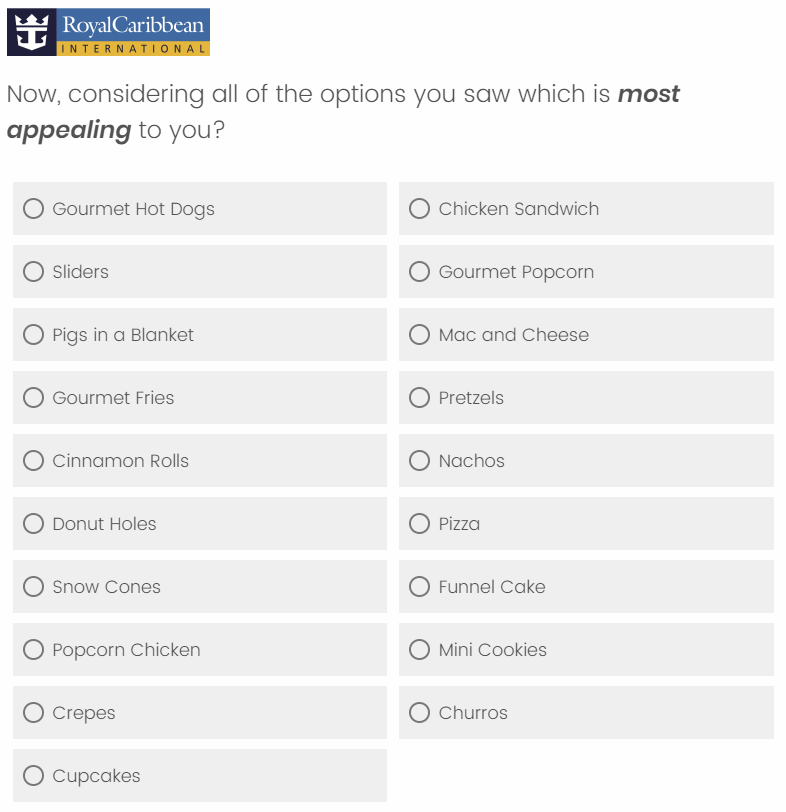An online survey question from Royal Caribbean, appearing on a stark white background with no borders. In the upper left corner of the image, the Royal Caribbean logo is displayed, comprising a black square with a white crown image on the left and a light blue rectangle with "Royal Caribbean" in white text situated above a gold strip with "INTERNATIONAL" in black, all in a landscape orientation.

The survey question is distinctly formatted and reads: "Now, considering all of the options you saw, which is most appealing to you?" with "most appealing" in bold italics and a line break after "most." Below this, the survey responses are organized into two columns against a dark gray background, each stretching horizontally longer than they are tall. 

On the left column, there are 10 options, each accompanied by an empty black circle for selection:
1. Gourmet hot dogs
2. Sliders
3. Pigs in a blanket
4. Gourmet fries
5. Cinnamon rolls
6. Donut holes
7. Snow cones
8. Popcorn chicken
9. Crepes (note: without an accent)
10. Cupcakes

The right column has 9 options:
1. Chicken sandwich
2. Gourmet popcorn
3. Mac and cheese
4. Soft pretzels
5. Nachos
6. Pizza
7. Funnel cake
8. Mini cookies
9. Churros

At the bottom, there's an empty white space on the right side where the tenth option would be if it existed. All selection circles are currently empty, indicating no answers have been selected yet.